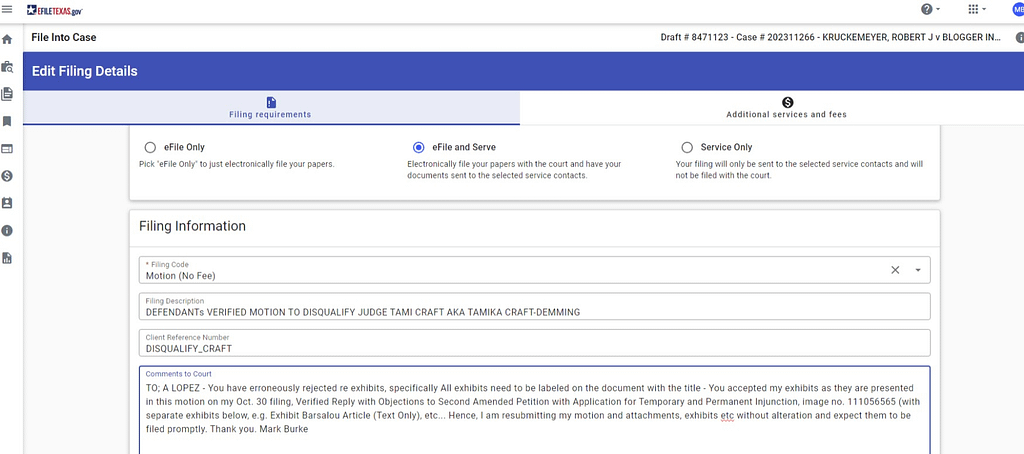Here is a cleaned-up and detailed caption for the image:

---

The image is a screenshot of the eFileTexas.gov website. At the top of the webpage, the logo consists of a blue box with a white star, and the heading reads "eFileTexas.gov." On the right side of the header, there is a gray circle featuring a question mark alongside a down arrow, a grid of nine dots (arranged in a 3x3 format) with a down arrow, and a blue circle that appears to contain the partially cut-off initials "MR."

The left sidebar includes a home button and several other symbols such as a dollar sign and a person icon, along with others.

The main section of the webpage is titled "File Into Case," followed by "Draft #8471123" and "Case #202311266." The case details indicate "Krueckemeyer Robert J versus Blogger In...," but the text is cut off. 

Underneath this heading, there is an option to "Edit Filing Details," which splits into two selectable choices: "Filing Requirements" and "Additional Services and Fees." "Filing Requirements" is currently selected.

Under "Filing Requirements," three options are visible: "e-file only," "e-file and serve," and "service only." The option "e-file and serve" is selected.

Next, in the "Filing Information" section, there are four fillable fields with the following details:
1. Filing Code: "Motion, No Fee."
2. Filing Description: "Defendant's verified motion to disqualify Judge Tammy Kraft, also known as Tamika Kraft Deming."
3. Client Reference Number: "Disqualify_Kraft."
4. Comments to Court: "To A. Lopez, you have erroneously rejected the filing regarding exhibits. Specifically, all exhibits needed to be labeled on the documents with the title. Thank you, Mark Burke."

Additional case information is likely present but not fully visible in the screenshot.